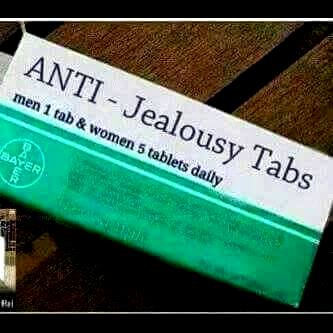This color photograph, presented in a square format with black stripes at the top and bottom, features a cleverly designed package meant to resemble a box of pills. The package, positioned diagonally from the top left to the bottom right corner, is predominantly white on the upper half and teal-green on the lower half, with a humorous label in black text. The label reads "ANTI-JEALOUSY TABS," with instructions below that state "Men: one tab, Women: five tabs daily," highlighting its gag gift nature. The top part text is in a typed font, with "ANTI" notably in all caps. The bottom left corner of the package displays a faux Bayer logo over the green background, adding to the mimicry of a real medication. This satirical item rests on a dark brown wooden surface, emphasizing the understated yet realistic style of the photograph.